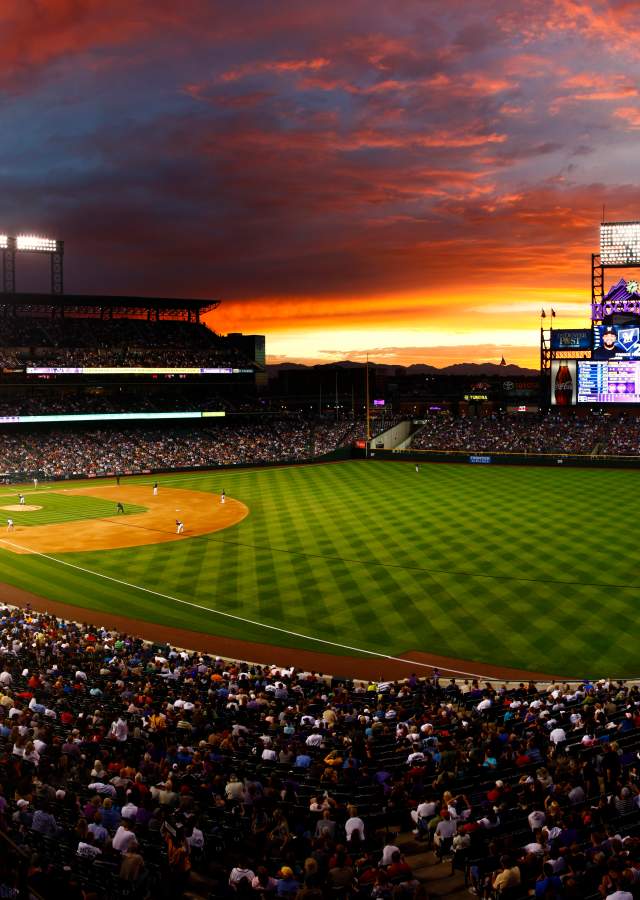This image captures a dynamic baseball game at a packed stadium, taken from a high vantage point during sunset or early evening. The sky is ablaze with hues of orange, red, yellow, and dark blue, punctuated by ominous clouds hinting at an approaching storm. The lush green field, meticulously patterned, occupies the center of the photo, with the baseball diamond prominently positioned towards the left. Surrounding the field are densely packed stadium seats filled with indistinct figures, casting shadows due to the stadium lighting. Prominent billboards in the background display player stats and a notable Coca-Cola advertisement. The LED scoreboards, though not clearly legible, add to the high-energy atmosphere of the game, enhanced by the visible sections leading to higher seating levels and the bright lights illuminating the field amidst the encroaching twilight.